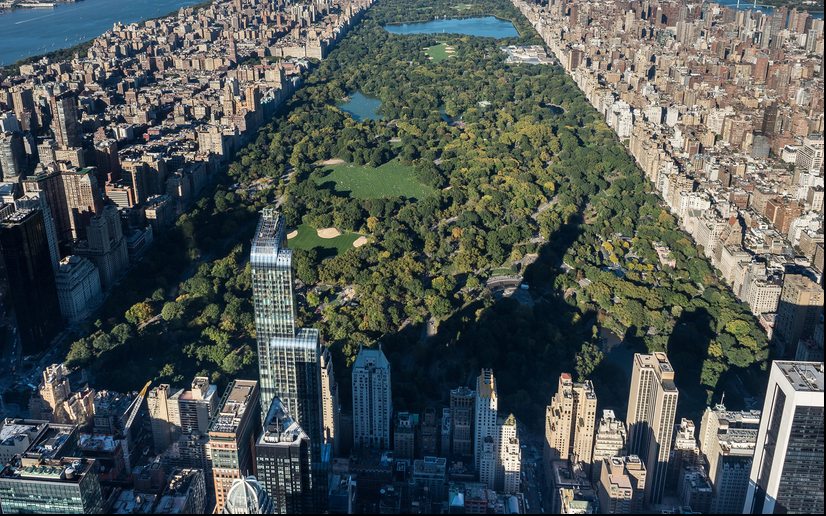This aerial daytime photo captures Central Park in New York City from the vantage point of one of its short ends. The rectangular park, dense with lush greenery and trees, is prominently punctuated by two large man-made ponds. Surrounded by towering skyscrapers and high-rises, the park stands out as a verdant oasis amidst the gray and brown urban landscape of buildings. The park extends vertically from the bottom to the top of the image, with the left and right sides bordered by tall buildings casting shadows into the park, suggesting it’s likely sunrise. Additionally, a significant body of water frames the city on the left side, further highlighting the juxtaposition between the natural beauty of Central Park and the dense urban environment that encloses it.